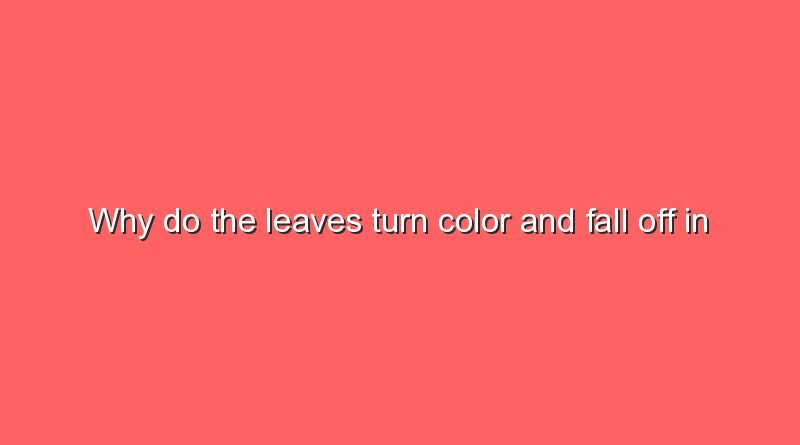The image depicts a salmon-colored horizontal rectangle with a solid background, roughly in a 16:9 aspect ratio. Centered perfectly within the rectangle is a single line of white text with a subtle black shadow, giving it a slightly raised appearance. The text reads, "Why do the leaves turn color and fall off in?" with a capital "W" at the beginning and the rest of the letters in lowercase. Notably, the text is an incomplete question that ends abruptly without punctuation, leaving the query unresolved.